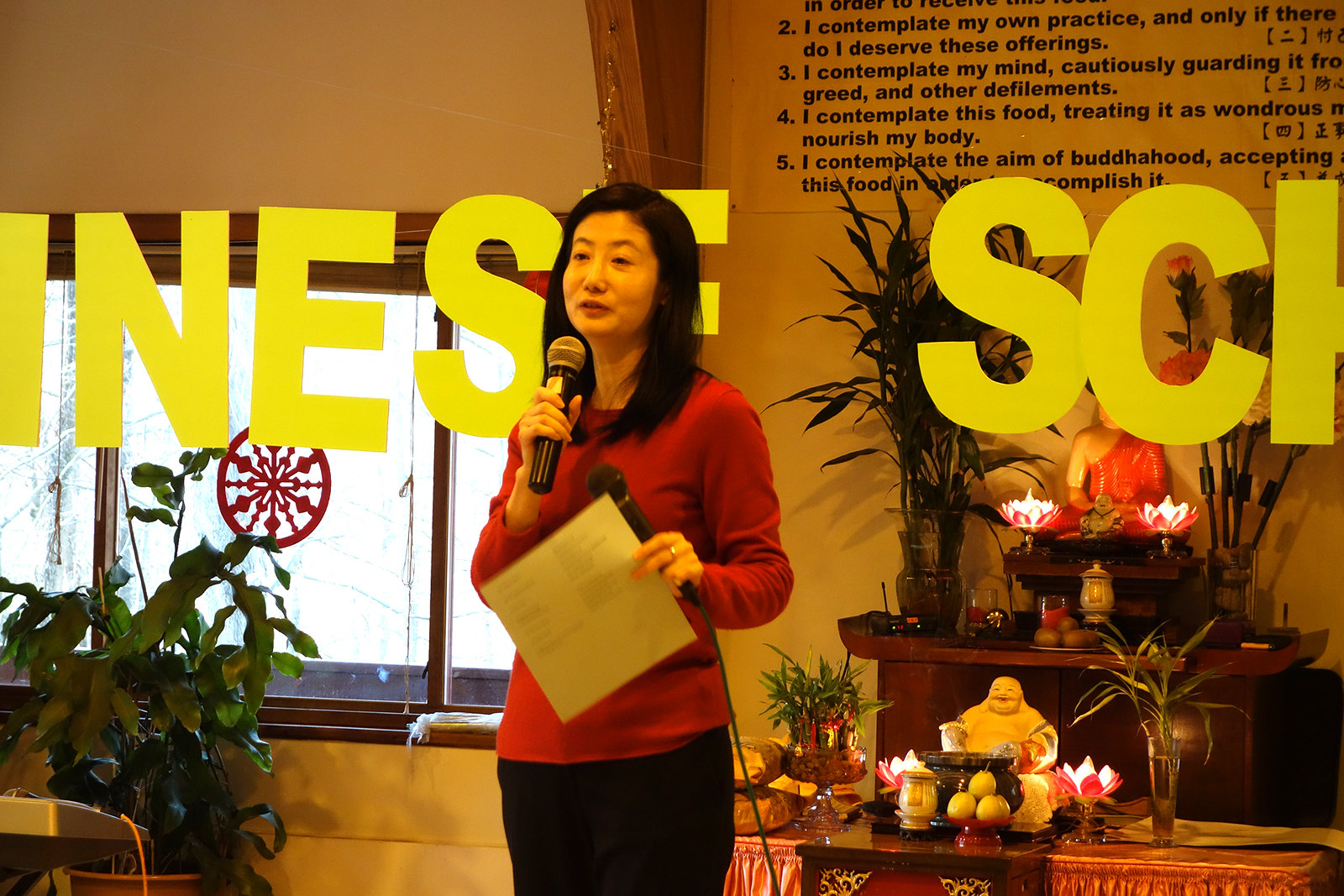In the image, an Asian woman with a long-sleeve red shirt and black pants is captured mid-speech, holding a wireless microphone in her right hand and a wired one in her left. In addition, she clutches a white sheet of paper. She stands before a slightly yellow-gray wall adorned with a poster that carries several Buddhist proverbs, including lines like, "I contemplate my own practice and only if there do I deserve these offerings," and "I contemplate this food, treating it as wondrous nourishment for my body." Further text discusses contemplating one's mind and the aim of Buddhahood. Large, partially obscured letters hang on thin strings behind her, spelling out "INESC" and hinting at a partially hidden word, possibly related to "school." The setting includes an altar with Buddha statues, flowers, and candles, adding to the contemplative and serene atmosphere.